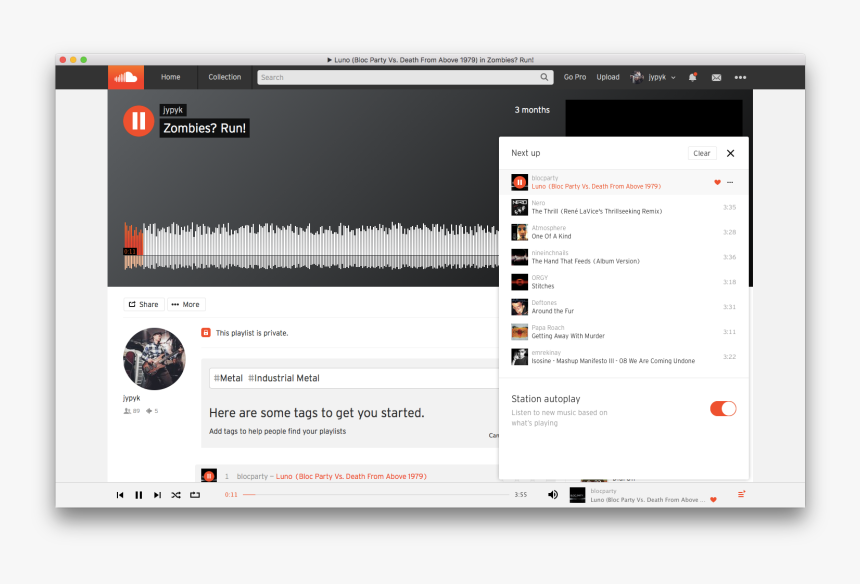Screenshot of the SoundCloud website displayed on a Mac desktop version browser. The distinctive red, yellow, and green circles at the top left signify it’s a Mac device. The screenshot captures the typical web page layout with a central address bar. The background is a light gray hue. At the top of the page, a black navigation bar spans across with the prominent SoundCloud logo—featuring an orange background and white cloud—on the left. To the right of the logo are two tabs, followed by a central search bar and more tabs on the far right. Below, the screen shows a song titled "Zombies? Run" currently playing, with the progress bar, or sound wave bar, barely progressed, indicating the song has just started. Additionally, there's a "Next up" section suggesting the upcoming songs in a playlist on the right.